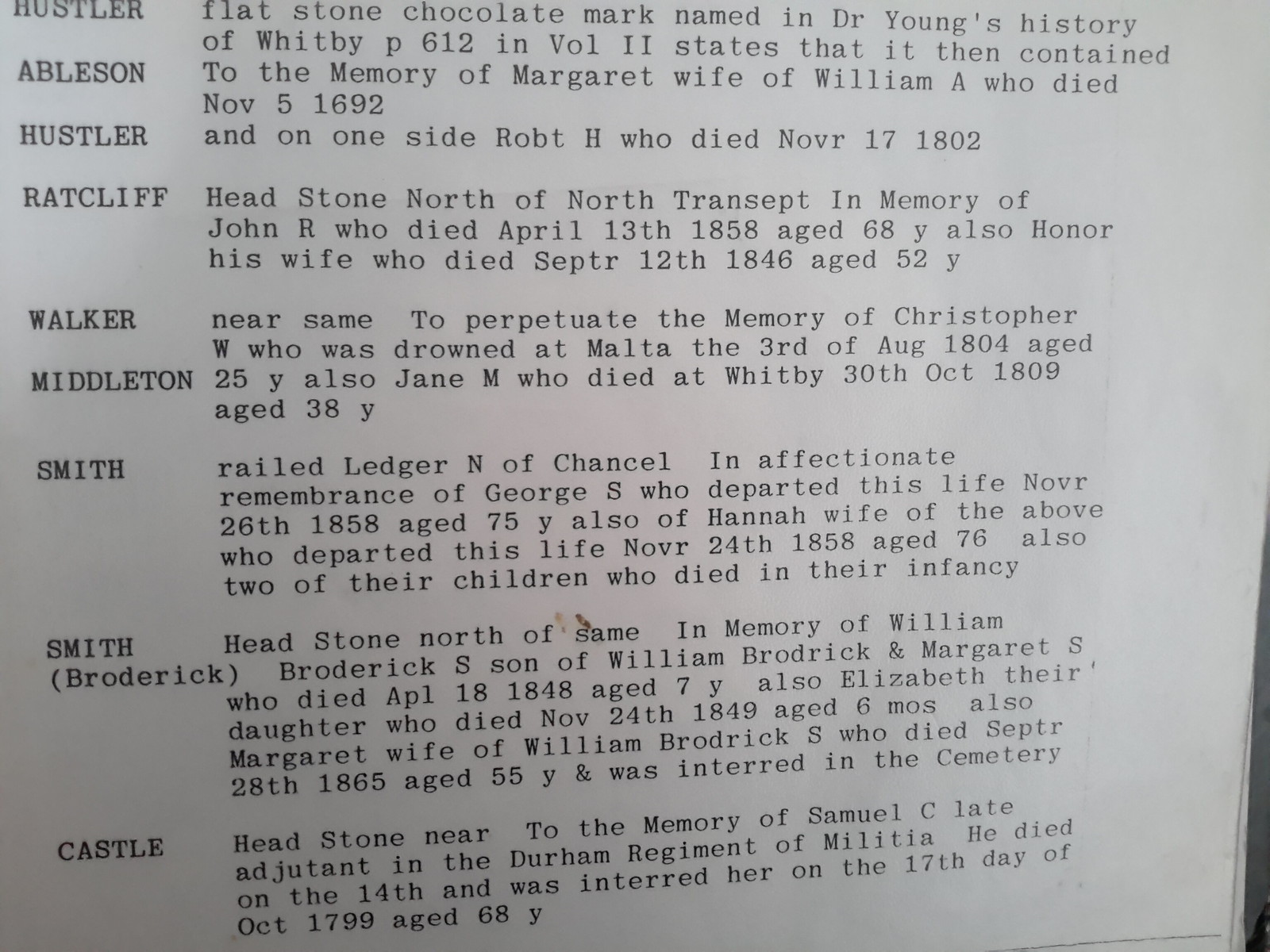The black and white image appears to be a detailed printed listing of various headstones in a graveyard, along with people memorialized on those stones, taken from historical records. At the top of the sheet, it mentions the word "Hustler," which is linked to several names throughout the document. The list follows a pattern with a column of names and associated paragraphs providing detailed descriptions on the right.

For instance, under the "Hustler" heading, it mentions a "flat stone chocolate mark" found in Dr. Young's History of Whitby, page 612, volume 2. Following this, "Abelson" relates to the memory of Margaret, wife of William A., who died on November 5, 1692. This pattern continues with entries like "Ratcliffe," which refers to a headstone north of the North Transept, in memory of John R., who died April 13, 1858, at the age of 68 years, as well as his wife who died on September 12, 1846, at the age of 52 years.

The document also mentions "Walker," with a record of a headstone near the same area to perpetuate the memory of Christopher W., who drowned at Malta on August 3, 1804, aged 25 years, and Jane M., who died at Whitby on October 30, 1809, aged 38 years. Entries for "Smith" record several individuals, including George S., who died November 26, 1858, aged 75 years, and his wife Hannah, along with two of their children who died in infancy.

Additionally, "Broderick" details a headstone north of the same area in memory of William Broderick S., son of William Broderick and Margaret S., who died April 18, 1848, at age 7 years, among others. Finally, "Castle" refers to a headstone near the memory of Samuel C., a late adjutant in the Durham Regiment of Militia, who died on October 14 and was interred on October 17, 1799, at age 68 years.

This document appears to function as a historical record, showing a list of names, their associated inscriptions, and details about their deaths and memorials, drawing from historical sources to provide a comprehensive overview of specific graves.